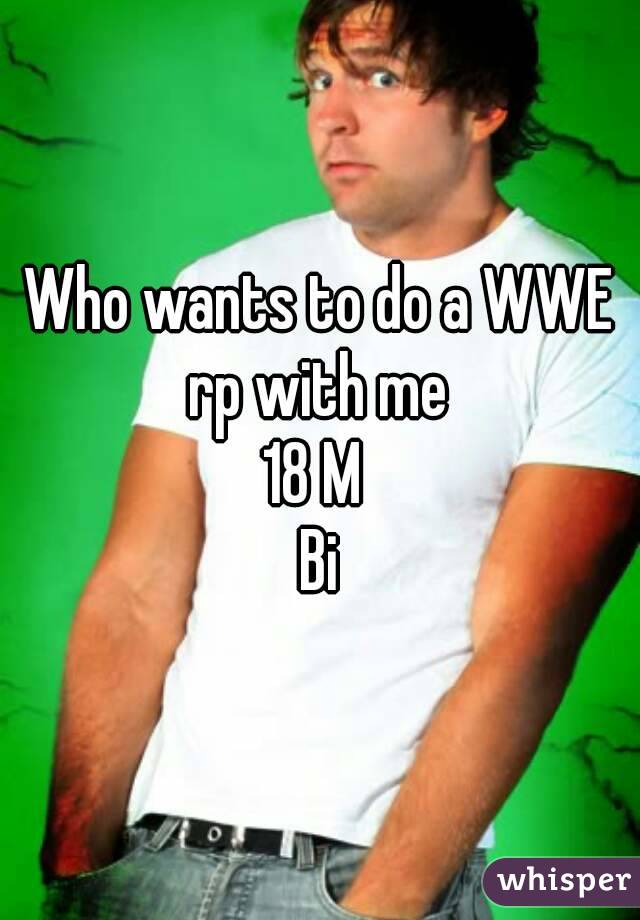The image features a young white male, likely in his 20s, with shaggy brown hair, standing upright against a solid green background with dark cracks. He is dressed in a white t-shirt, a black belt, and blue jeans, with his hands casually placed in his pockets. His face bears a surprised or anxious expression as he looks directly at the camera, his body turned slightly to the left. Overlaid on the photo in white font, it reads: "Who wants to do a WWE RP with me? 18M. Bi." In the bottom right corner of the image, there is a dark purple oval containing the word "Whisper" in white font.